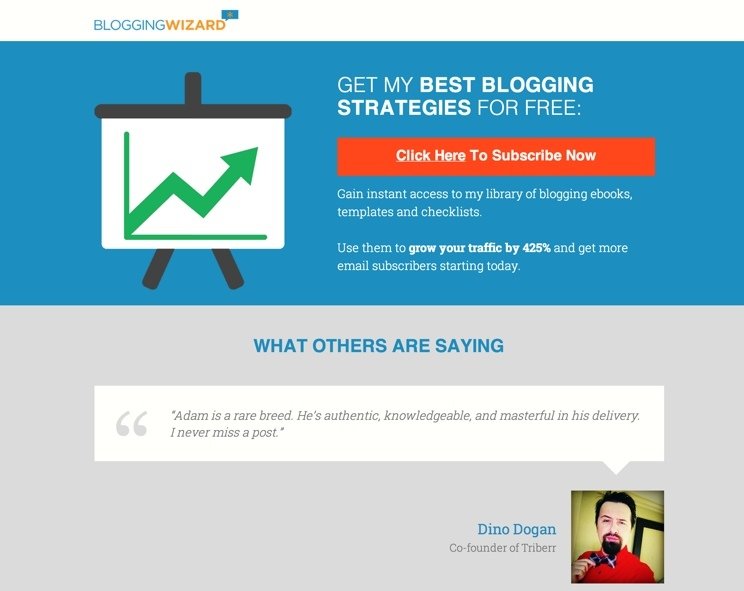Screenshot of the Blogging Wizard Website App

The screenshot captures the web page of the Blogging Wizard website app. At the top of the page, the app's name is prominently displayed: "Blogging Wizard" — with "Blogging" in blue and "Wizard" in yellow.

The content is divided into two primary sections. The upper section has a blue background with a bold title: "Get my best blogging strategies for free." This is followed by a striking red button that reads: "Click here to subscribe now." Below the button, the text offers enticing details: "Gain instant access to my library of blogging eBooks, templates, and checklists. Use them to grow your traffic by 425% and get more email subscribers starting today."

The lower section, set against a gray background, is titled "What others are saying." Here, a profile picture of Dino Dogan, identified as the co-founder of Triberr, is displayed. Under his image, a glowing testimonial reads: "Adam is a rare breed. He's authentic, knowledgeable, and masterful in his delivery. I never miss a post."